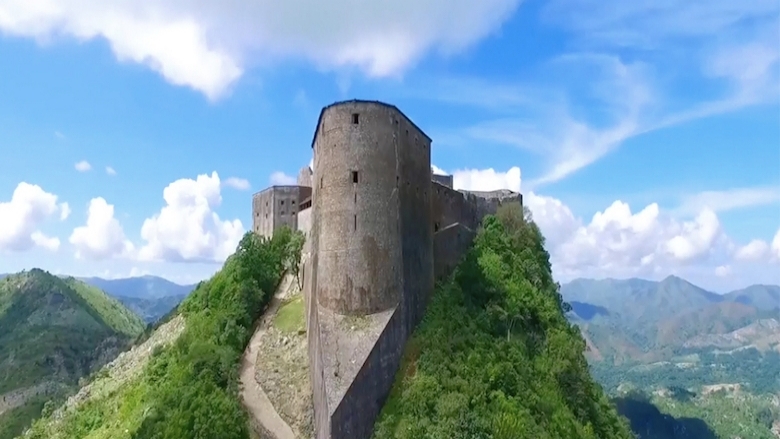The image showcases a majestic, older-style castle, constructed from gray stone, perched precariously at the very peak of a steep cliff. The castle features a prominent triangular-shaped structure at its base, designed to make the ascent challenging for potential attackers, and a towering structure that enhances its formidable appearance. Small windows punctuate the castle’s walls, which extend near the cliff’s edge, highlighting its strategic defensive position. 

A narrow path winds its way up the cliffside, providing the only accessible route to the castle, further emphasizing its fortified nature. Surrounding the imposing structure are lush trees and greenery, blending into the mountain landscape. In the distance, a panorama of gray and green mountains stretches out under a bright blue sky adorned with swirling white clouds. This aerial photograph, likely captured with a drone, captures the scene in vivid detail, showcasing the castle’s dominance over the surrounding natural terrain at this mountain's summit. The setting is illuminated by ample natural daylight, contributing to a clear and vibrant depiction of this imposing fortress.